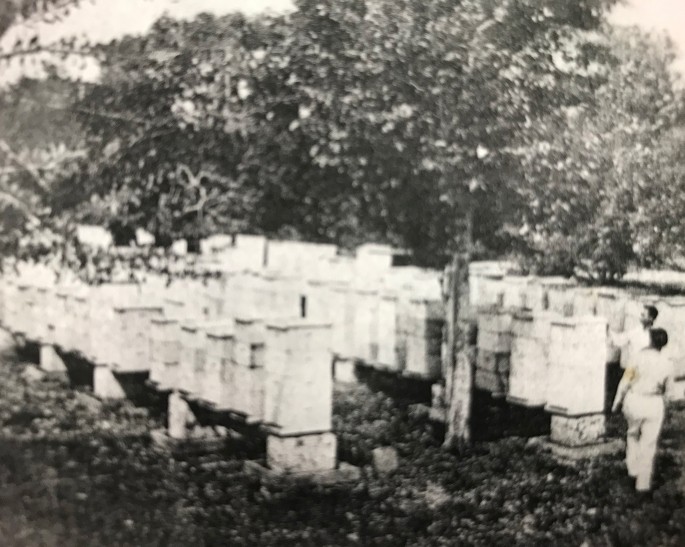In this square black-and-white photo, the image is blurry and grainy with no border or text. The top portion shows a canopy of tree leaves and a pale sky peeking through the upper left and right corners. The overall coloration appears as shades of light brownish white. The center of the photograph features numerous vertical rectangular structures – potentially rows of stones that might resemble gravestones but don’t clearly indicate a cemetery. These structures are arranged visibly in rows, particularly noted on the left side where one stands at a diagonal position. Between these rows, two figures, a man and a woman, stand on the right side. The man is seen touching the ends of one of these rows, while the woman is dressed in pants and a shirt. The man’s shirt is visible, though other details are obscured. Surrounding this scene, the ground displays a mix of brownish-black shades suggestive of grass and leaves. Trees and additional foliage backdrop these structures and individuals, giving a sense of an outdoor setting with an uncertain purpose for the mysterious, tall, and thin rectangular objects scattered throughout the image.